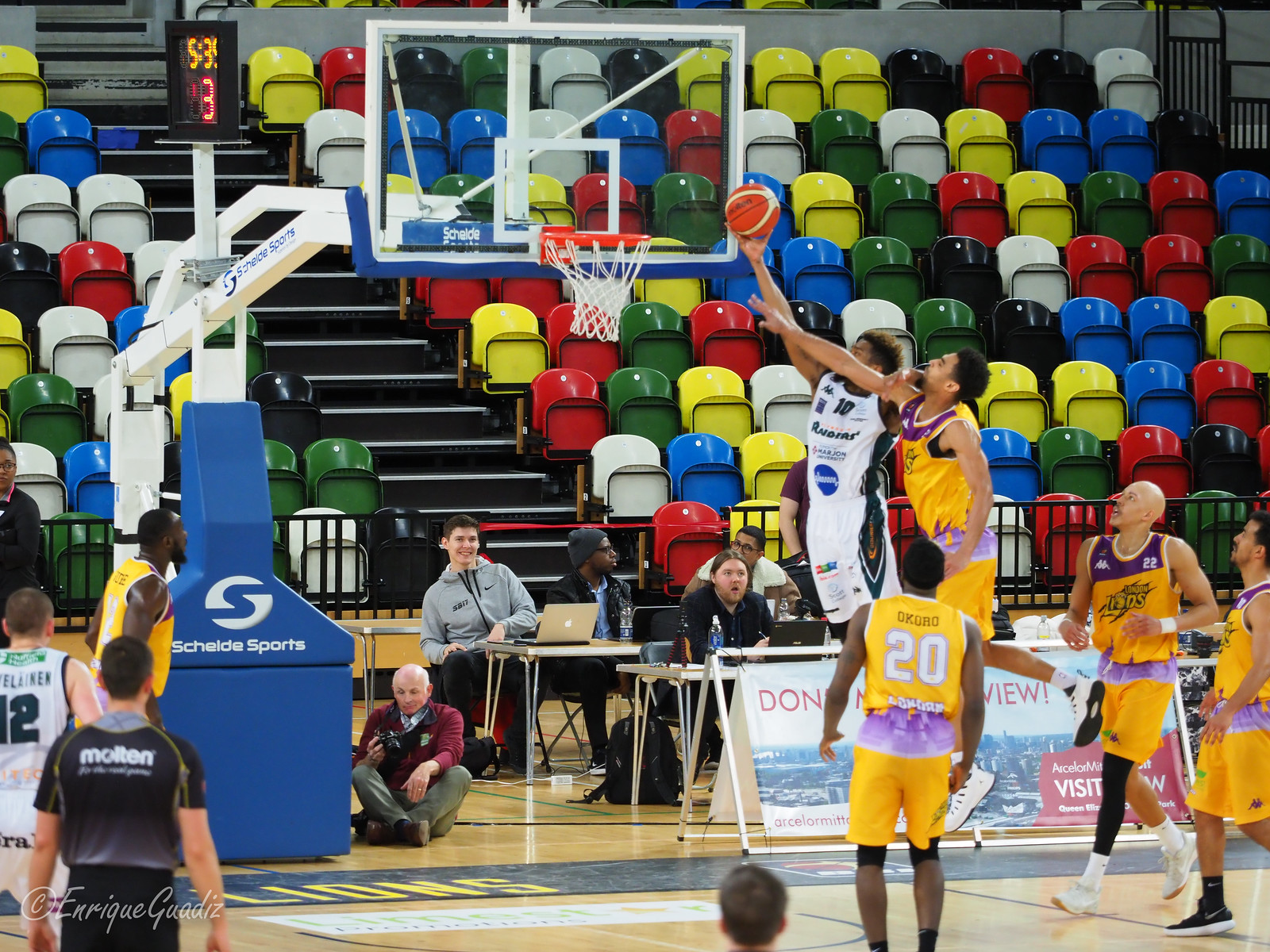This detailed image showcases a vibrant scene on an indoor basketball court during what seems to be a festival or exhibition game. Center stage are five basketball players: four wearing yellow and purple jerseys and one in a mainly white jersey. The action focuses on the player in white attempting a basket while a yellow and purple-clad opponent leaps to block the shot. 

On the ground, three more players in yellow and purple are positioned on the right, while one player from each team can be seen on the lower left. A referee and a photographer, who is sitting near the stand marked "Seidi Sports" with its logo and some timing equipment showing "5:35" and a red "3," are also part of the busy scene. 

The background features an array of brightly colored seats in red, black, green, blue, yellow, and white, evoking a playful, almost elementary school-like atmosphere. Near the table set along the sidelines, people are engaged with several laptops, alongside a water bottle, continuing the dynamic and lively ambiance of the scene.